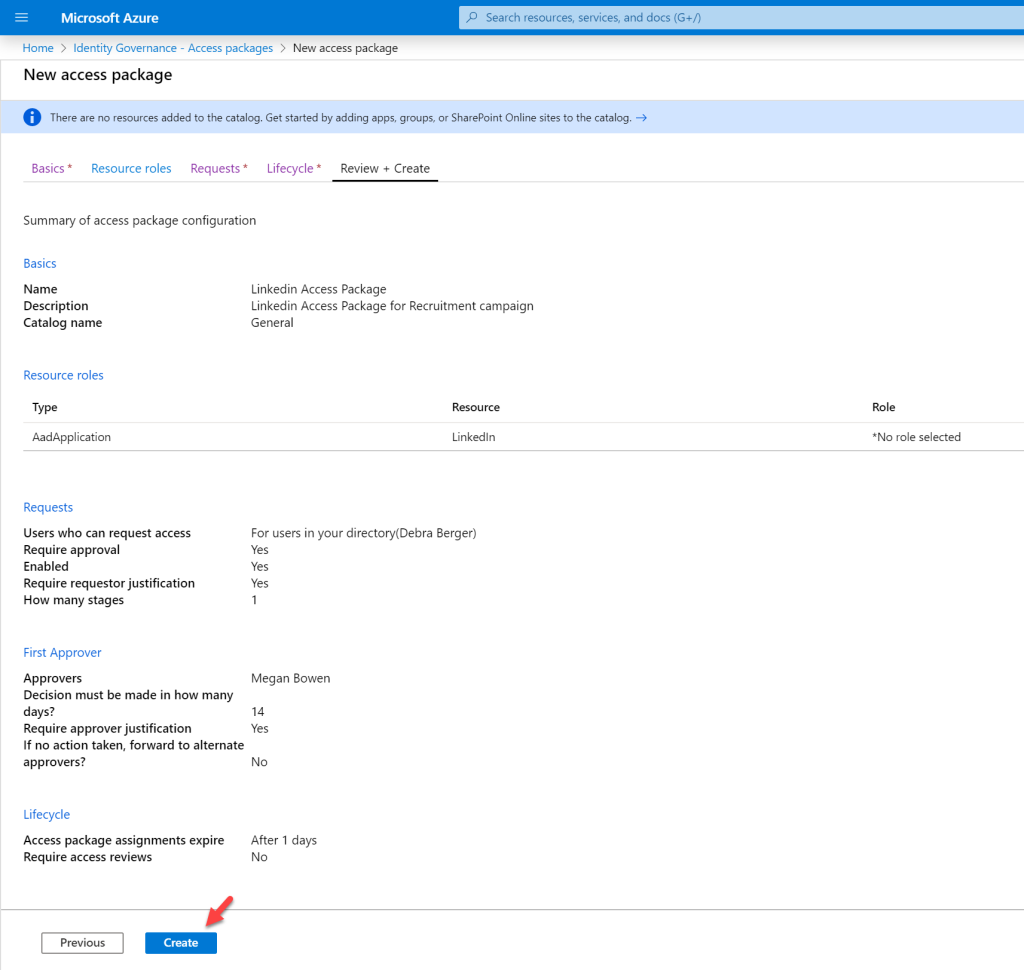Sure, here's a detailed and cleaned-up caption based on the provided description:

---

**Detailed Description of Microsoft Azure Interface for Access Package Configuration**

The interface on the Microsoft Azure portal features a blue background. On the top left, there's a settings icon, and on the top right, a search bar allowing users to search for resources, services, and documents. 

Below the top navigation, on the left-hand side, the home tab is displayed along with a tab labeled "Identity Governance." Within this tab, the user is focused on "Access Packages" and specifically on creating a "New Access Package," shown in bold, large text.

The main body of the interface states: "There are no resources added to this catalog. Get started by adding apps, groups, or SharePoint Online sites to the catalog." An information icon (a lowercase 'i' inside a circle) appears to the left of this message.

The interface showcases different sections in a step-by-step manner, with sections titled "Basics" (highlighted in purple with asterisks), "Resource roles" (in blue), "Request," and "Lifecycle." The current focused section is "Review + Create."

Towards the bottom, a summary lists the configuration details of the access package:
- **Name:** LinkedIn Access
- **Description:** For recruitment campaign
- **Catalog Name:** General Category

In the "Resource Role" section, details are provided:
- **Type:** AAD Application
- **Resource:** LinkedIn
- **Role:** No role

In the "Request" section, the following information is displayed:
- **User can request access for your directory:** According to Debra Berger
- **Required approval:** Yes
- **Enabled:** Yes
- **Required requestor:** Yes
- **Number of stages:** Only one
- **First approver:** Megan Bowen, with a decision required within 14 days
- **Required approver justification:** Yes
- **No alternate approver specified**

In the "Lifecycle" section:
- **Expiration:** After one day
- **Silence expiration:** Yes
- **Requires access reviews:** No

At the bottom of the configuration pane, there are two buttons: a "Previous" button in white, and a "Create" button in blue, with an arrow pointing toward the "Create" button.

---

This provides a clarified, detailed view of the interface described for the Microsoft Azure Access Package configuration.